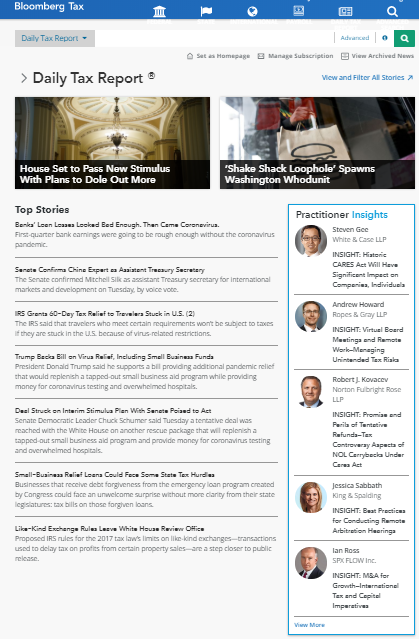In the top left corner of this image, various headlines and news snippets from Bloomberg Tax's Daily Tax Report are prominently displayed. The main headline discusses the proposal of a new stimulus package and plans to distribute additional funds, drawing attention to a related article on Shake Shack's exploitation of loopholes and its ramifications in Washington. The image also highlights job stories and the financial implications of the coronavirus pandemic on banks, specifically concerning loan losses anticipated in the first quarter earnings even before the pandemic exacerbated the situation.

A notable headline confirms the Senate's approval of Mitchell Silk as Assistant Treasury Secretary for International Markets and Development, completed by a voice vote on Tuesday. Additionally, an IRS announcement provides a 60-day tax relief for travelers stranded in the U.S. due to virus-related restrictions, stipulating that those who meet specific criteria will not be subjected to taxes under these extraordinary circumstances.